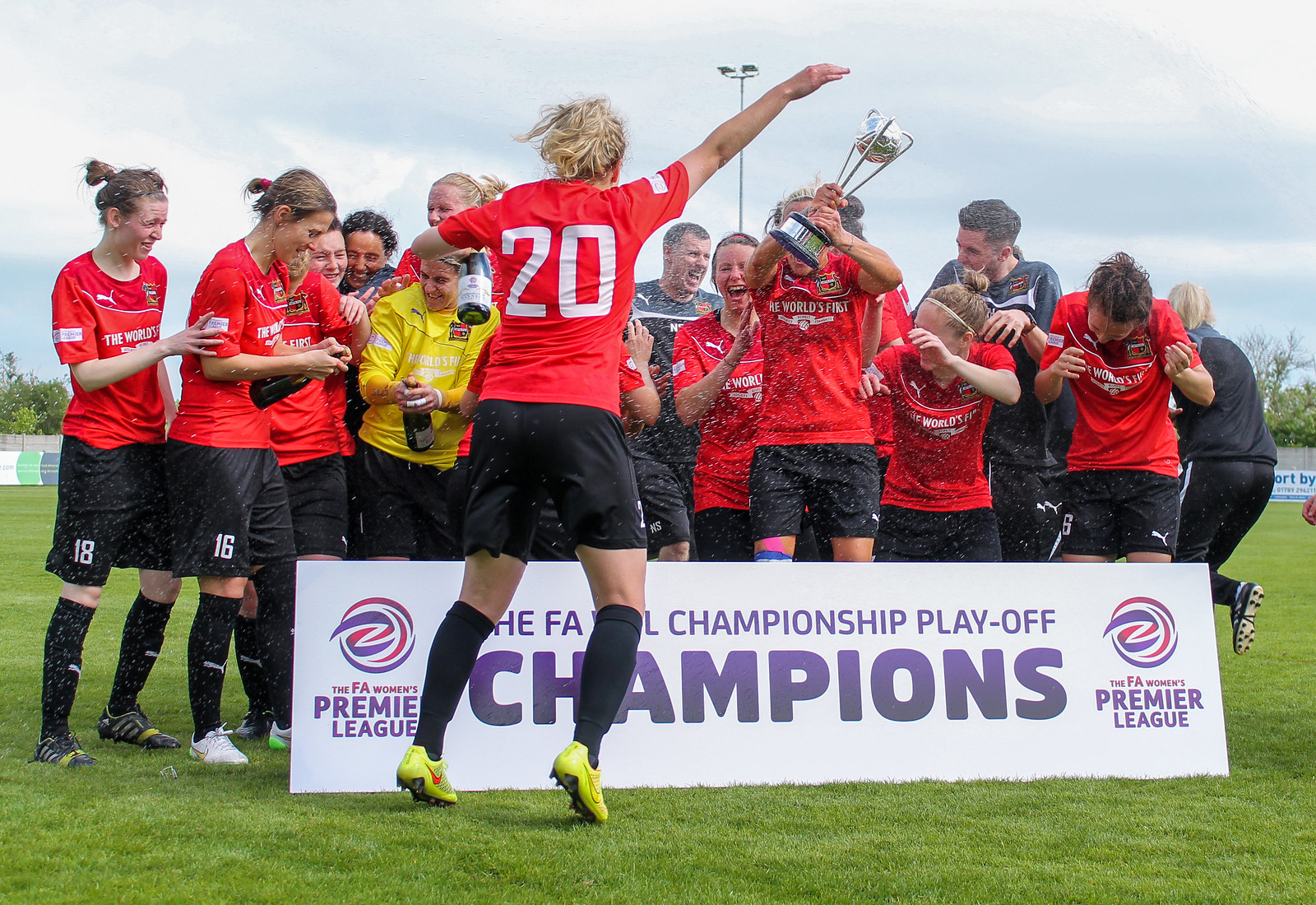In this vibrant image, a women's soccer team is exuberantly celebrating their championship victory on a lush green soccer field under a clear blue sky with a few scattered clouds. The team is dressed uniformly in red short-sleeved jerseys with white numbers, black soccer shorts, and black socks bearing a white Puma logo. The central figure, player number 20, with blonde hair, is energetically jumping and raising her right hand while holding a champagne bottle in her left.

The scene is dominated by a prominent white placard with bold purple lettering that reads, "FA Women's Premier League Championship Playoff Champions." To the left of this placard, players number 18 and 16 can be seen, while to the right, a group of five players is partially obscured, with the one in front proudly hoisting a silver trophy with a soccer ball atop.

Surrounding the jubilant players are their coaching staff, including an older male coach dressed in black and a female coach in a yellow long-sleeved shirt, who is also holding champagne. The celebratory mood is palpable, with champagne flying through the air, marking a triumphant moment for the team as they revel in their hard-earned success amidst the sprawling, flat green field.